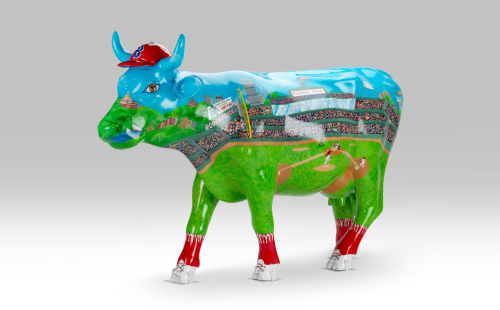This detailed landscape-oriented color photograph showcases a meticulously decorated bulls figure, seemingly ceramic, plastic, or paper mache, adorned with an intricate mural of Fenway Park, the iconic Boston Red Sox baseball park. The bull, actually a bull due to its prominent horns, wears a distinctive red baseball cap featuring the Boston "B." Its body is richly painted to depict the ballpark: the upper back and horns are blue, representing the sky, while the midsection showcases green grass field and brown dirt infield, with detailed spectator stands filled with fans and banners. The yellow foul pole is visible on its neck, and the park's players are depicted on the field. Adding to its thematic design, the bull's legs are painted as red socks with white cleats adorned with little red shoelaces. The background of the image transitions from a dark to light gray gradient, providing a neutral backdrop that emphasizes the vibrant realism of the bull's intricate Fenway Park mural.